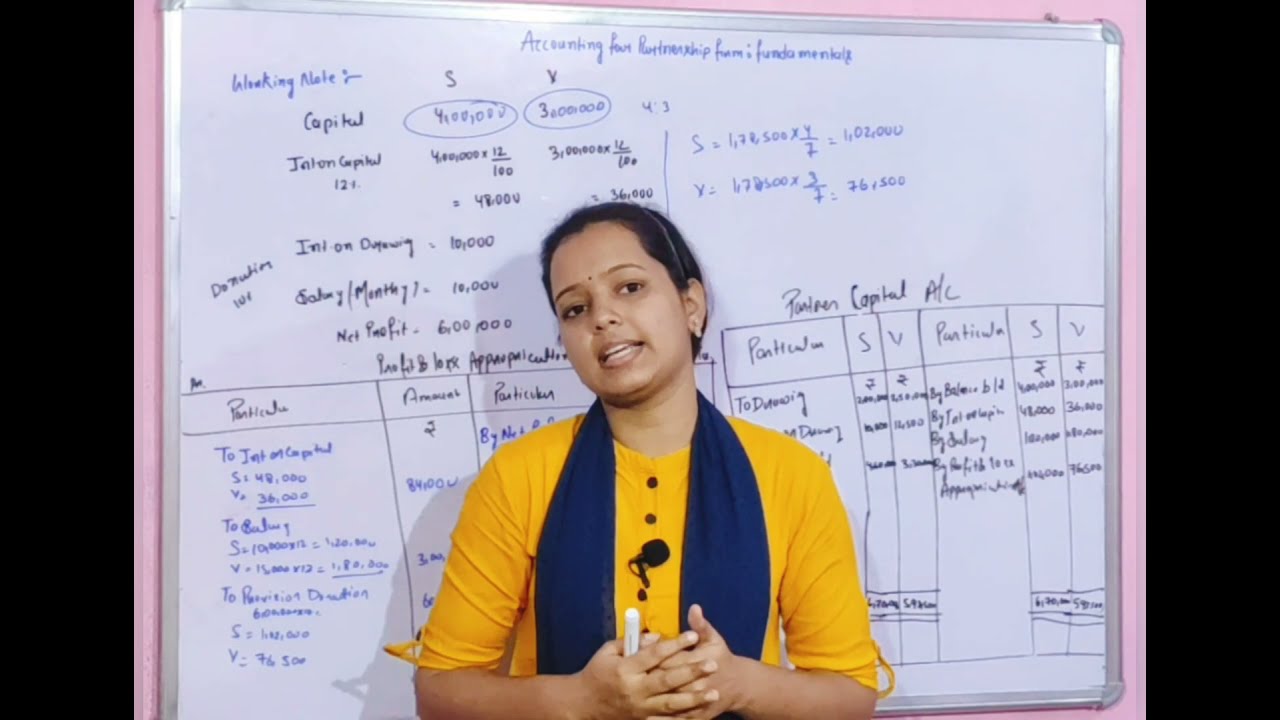This photograph depicts a young South Asian woman, potentially a professor or a teacher, standing indoors in front of a whiteboard that’s mounted on a pink wall, with black vertical strips on either side of the image. She is the focal point, positioned in the middle, and is gazing directly at the viewer while speaking. She has dark features, brown hair pulled back with a thin hairband, and a small dot between her eyebrows. She wears a bright yellow blouse with sleeves reaching to her elbows and a long, dark blue scarf draped around her neck. A black microphone is clipped to the button area of her blouse. Her hands are clasped together in front of her, holding a whiteboard marker. 

Behind her, the whiteboard is filled with text written in both black and blue markers. The top section, written in blue, includes the phrase "accounting for partnership form and fundamentals," although the handwriting can be challenging to read. Below this, numbers and equations are visible, including a table with rows and columns featuring data such as the word "CAPITAL" accompanied by figures like "four million" and "three million." The woman’s head is slightly tilted to the left, and she appears animated in her lecture, with her teeth showing as she speaks.